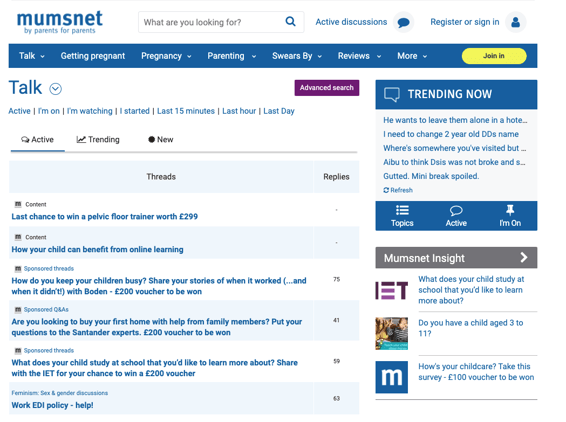This image is a detailed screenshot of a website, predominantly a white background, showcasing a parenting forum titled "Mumsnet" with the tagline "By parents, for parents" in blue text located in the top left corner. The upper section of the page features a comprehensive menu bar with a blue strip and white text, containing navigation options such as "Talk," "Getting Pregnant," "Pregnancy," "Parenting," "Swears By," "Reviews," and "More," alongside a prominent yellow "Join In" button. Below this menu bar, there’s a prominent search bar with the prompt, "What are you looking for?" and options for "Active discussions," "Register," and "Sign in."

The main section of the webpage, labeled "Talk," displays a variety of forum threads, with options for filtering posts by "Active," "I’m On," "I’m Watching," "I Started," and time frames like "Last 15 Minutes," "Last Hour," and "Last Day." Featured threads include sponsorships, community questions, and discussions, such as "Last chance to win a pelvic floor trainer worth £299," "How your child can benefit from online learning," and "How do you keep your children busy? Share your stories with Bowdoin for a chance to win a £200 voucher." 

On the right side of the page, there's a "Trending Now" section with popular posts and "Mumsnet Insight," featuring articles and surveys, including "How's your child care? Take this survey for a chance to win a £100 voucher" and details about school studies and parental concerns. The logo consists of the letter "M" and is prominently featured. The entire layout reflects a user-friendly message board designed for active parental engagement and community support.